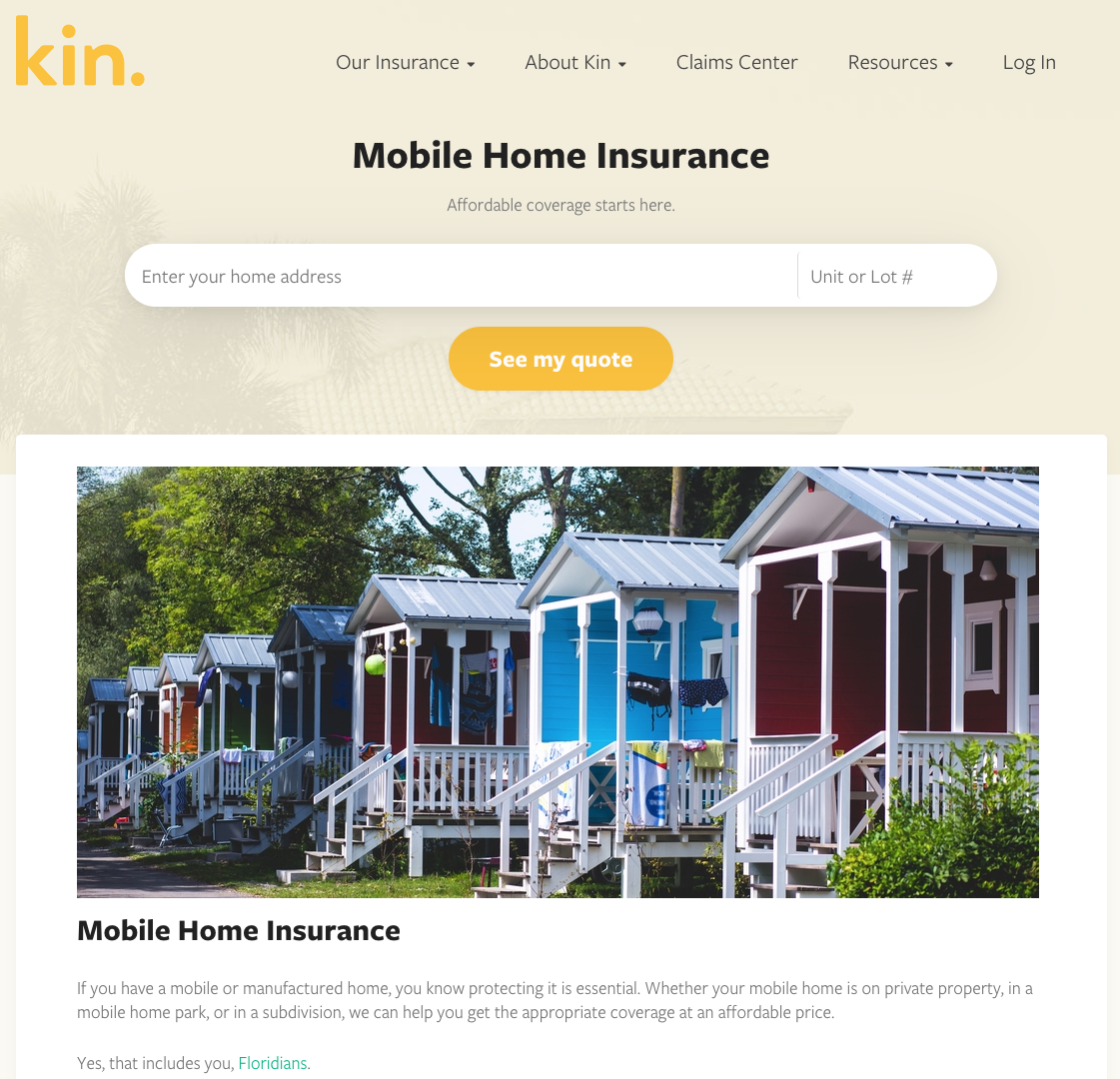The image is a screenshot from a website focused on mobile home insurance, specifically from a company called KIN, as indicated by the white text "KIN" at the top. The navigation bar at the top of the page features links to "Our Insurance," "About KIN," "Claims Center," "Resources," and an option to log in.

In the center of the page, the bold text "Mobile Home Insurance" stands out, with the tagline "Affordable coverage starts here" written in gray beneath it. The interface prompts users to enter their home address and unit or lot number.

A distinctive, slightly curved, yellowish-orange rectangle prominently displays the call-to-action button "See My Quote." Below this, a picture features several mobile homes aligned in a row, each with steps leading down to a sidewalk.

The accompanying text emphasizes the importance of protecting mobile or manufactured homes, whether they are located on private property, in a mobile home park, or in a subdivision. It reassures potential clients that the company can help secure affordable and appropriate coverage. The message particularly highlights that their services are inclusive of Floridians, with "Floridians" written in green text.